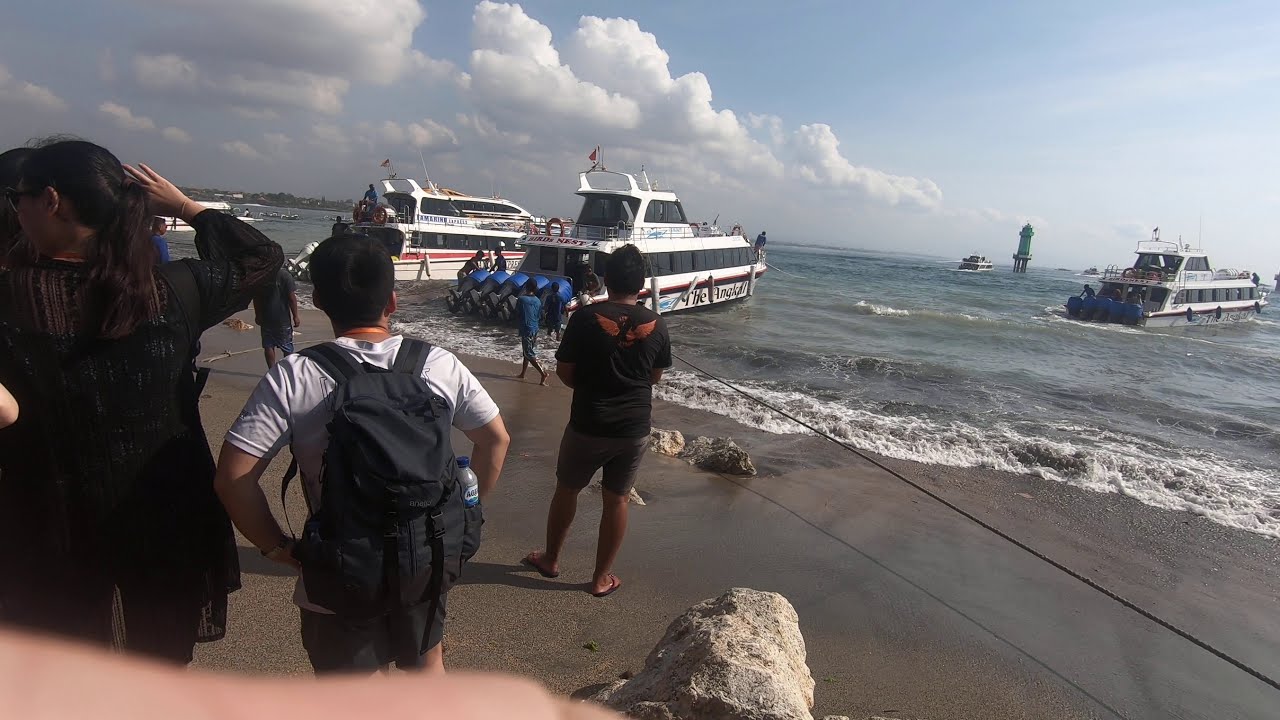The beach scene depicted shows several people, likely spectators, standing on the dark, dirty brown sand, some wearing backpacks, shorts, flip-flops, and black shirts. In front of them, waves ripple towards the shore from a body of water that transitions from greenish-gray near the beach to a darker blue further out. A prominent gray rock lies directly at the foreground's edge. In this water are multiple boats, including at least two large, white ferry boats near the shore, each with blue details at their backs. There is also a lighthouse on stilts visible in the middle distance of the water. Off farther into the distance, additional boats can be seen, possibly engaged in maintenance or other activities. The sky is a light blue, filled with an abundance of large, puffy white cumulus clouds, particularly concentrated in the upper left part of the image. A rope runs diagonally in front of one of the nearby men, stretching from the left side of the frame.